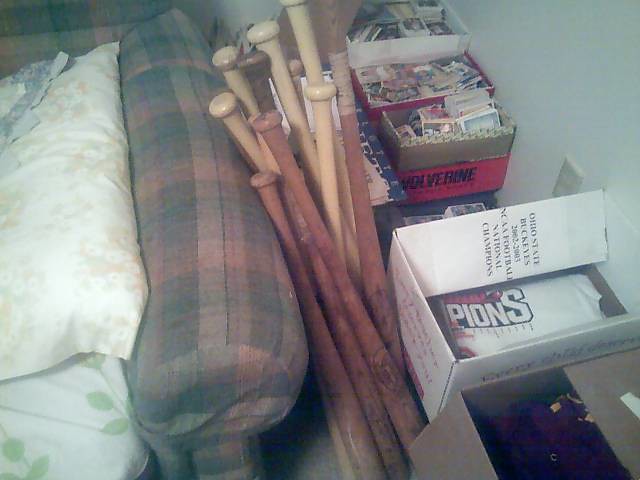This image captures the corner of a room dominated by a plaid couch in muted hues of blues, reds, and yellows. Positioned against the left arm of the couch are at least 11 wooden baseball bats with their handles up, showing signs of age and wear. Surrounding the bats is a mixture of cardboard boxes; the nearest one is dark inside, while another prominently reads "Pawnee" and appears to contain a t-shirt. Additional boxes, likely holding sports memorabilia and trading cards, are arranged to the right of the bats, with one particularly holding baseball cards. The room also features a grayish-white wall with a visible outlet, and white bed pillows propped against the couch. The overall scene suggests a collection of cherished sports items in an intimate, indoor setting.